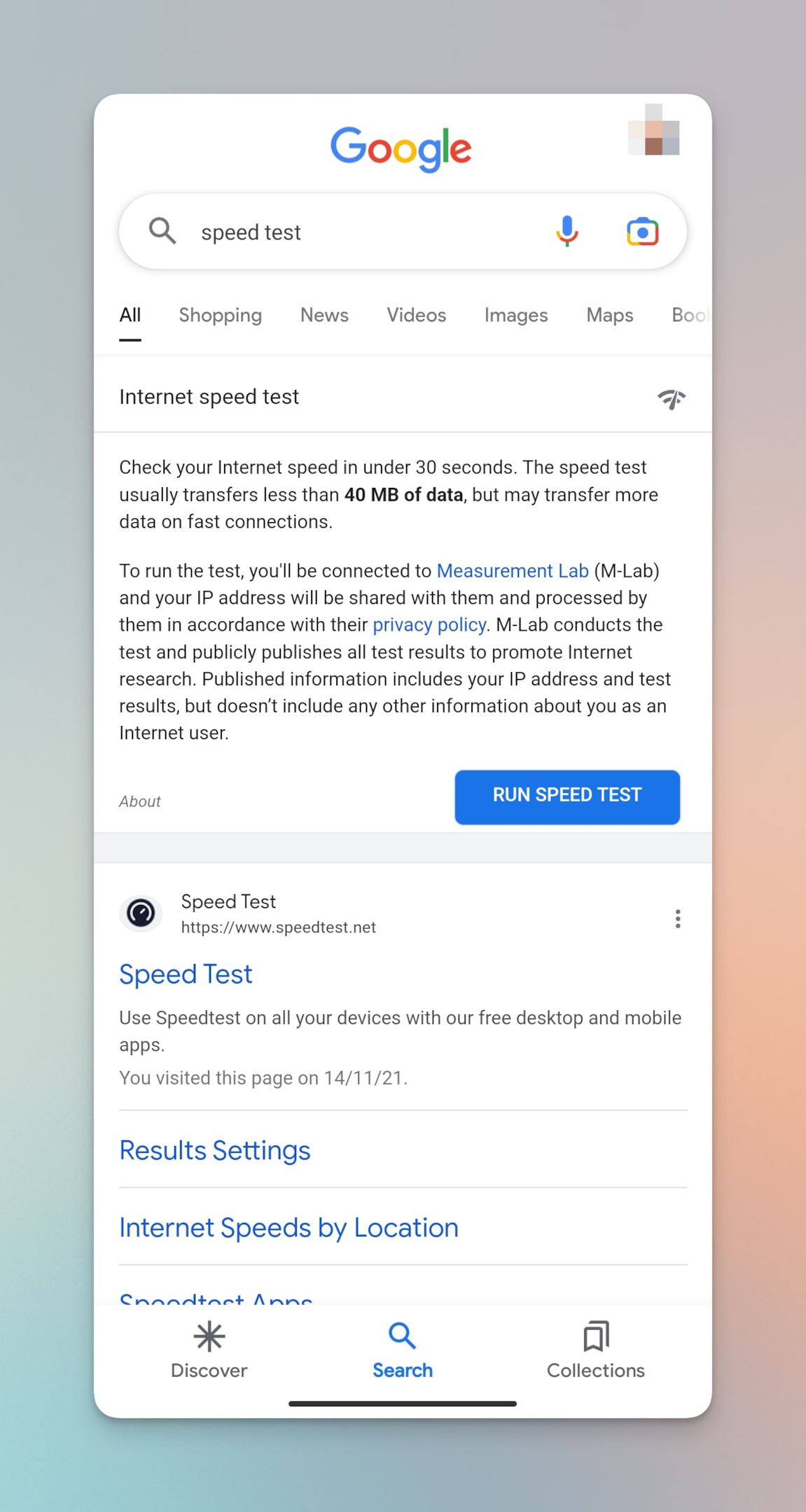The image appears to be a screenshot from a smartphone, characterized by its elongated vertical format, roughly three times longer than it is wide. The backdrop features a gradient, transitioning from a grayish-purplish hue encompassing the top inch, the left, right, and bottom edges, to a pinkish color about halfway down the right side extending to roughly two inches from the bottom.

Centered within this backdrop is the actual screenshot content. At the very top, there's a white bar displaying the Google logo, with the letters "G" in blue, "O" in red, "O" in yellow, "G" in blue, "L" in green, and "E" in red. To the right of the logo, there is a blurred-out section.

Directly beneath this, there is a search bar spanning the width of the screen, featuring a search icon on the left, the text "speed test" inside the bar, and a microphone icon and camera icon on the right.

Below the search bar, there are tabs with black text: "All" which is underlined with a thin black line, followed by "Shopping," "News," "Videos," "Images," "Maps," with the latter partially obscured.

In the main content area, titled "internet speeds", there's a Wi-Fi icon on the right, which is partially blocked out. Below this, a paragraph of three lines discusses internet speeds, followed by seven additional lines of supporting information.

Toward the deeper part of the screenshot, on the right side, there is a small blue tab with white text that reads "run speed test." Below it, there is a thin gray border enclosing more white space. Within this space, a small black icon with a lot of white lines appears, accompanied by the text "speed test" indicating the website, which also includes some information about the test. 

Underneath, smaller blue text reads "real results" and "settings," succeeded by a section titled "internet speeds by location" in blue.

At the very bottom, a navigation bar displays icons and text: an asterisk with "discover" beneath it, a search icon with "search" labeled in blue, and a collections icon labeled "collections."